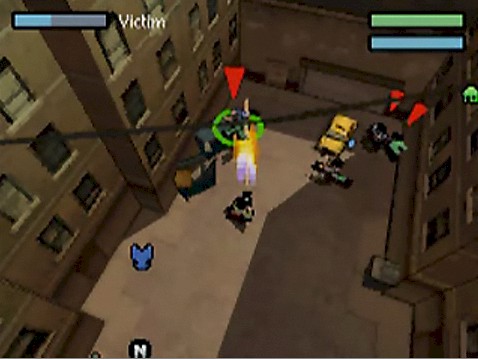This is a detailed screenshot from a video game depicting an overhead view of a city courtyard situated among high-rise brick apartment buildings. The buildings are brownish-tan with multiple windows, approximately five per story. The central communal area contains a yellow vehicle resembling a taxi or sports car, beside which there are avatars representing several game characters. Several shapes identified as people are marked by upside-down red triangles pointing towards them. Notably, one character is encircled by a green circle and labeled as the victim, hinted by the presence of a health bar in the upper left corner, which is partly light blue (40%) and gray (60%), accompanied by the word "victim" in white text.

In the top right corner, there are green and blue bars stacked horizontally like an equal sign. The scene shows indications of a conflict, with one character seemingly engaged in gunfire, represented by an orange-yellow muzzle flash. On the bottom left, there's a small blue bird icon, and in the very bottom of the screen, a black circle encloses the letter "N." Additionally, on the bottom right, there appears to be a grey box, possibly an AC unit or duct. The environment is further detailed by the presence of a grey platform area between the buildings and a garage door visible on the top right side of the image.